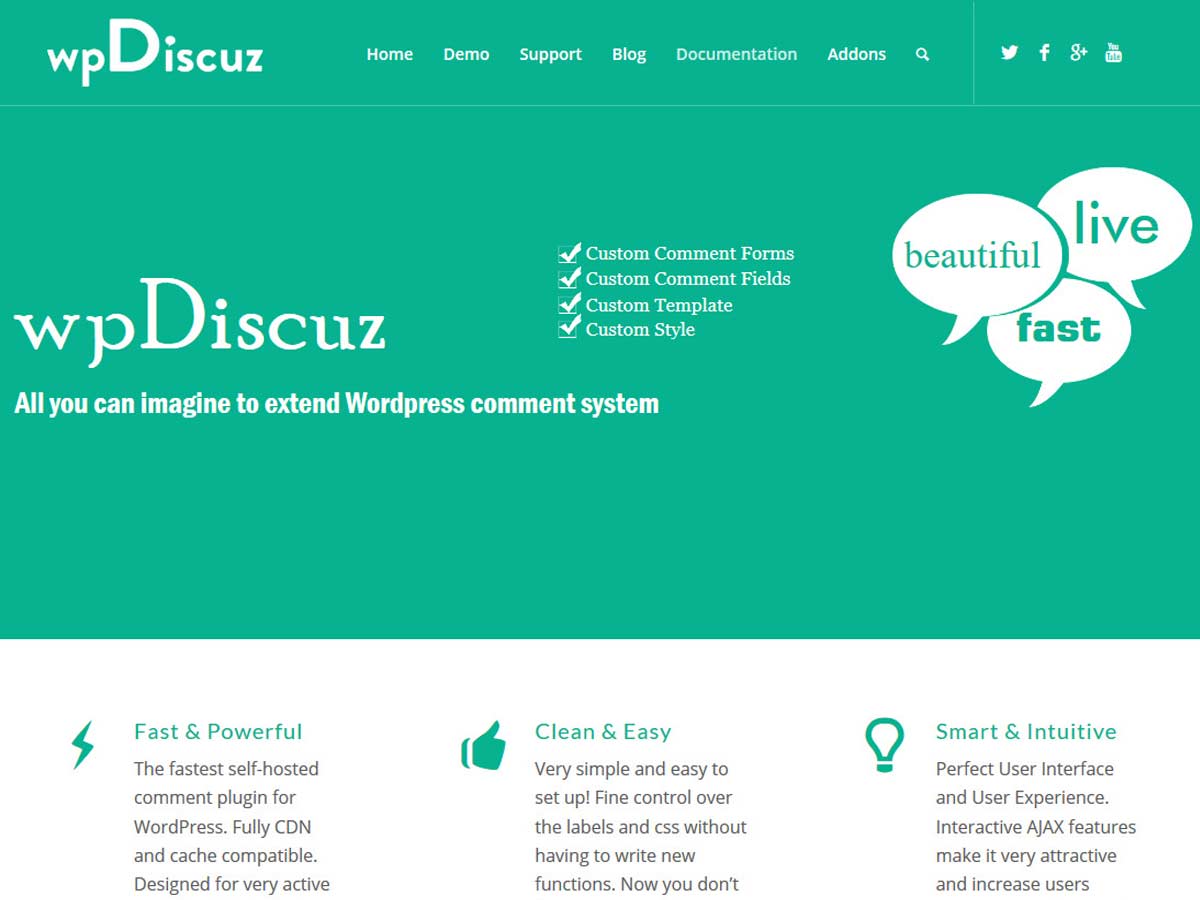A screenshot from the WPDiscuss website features a serene, mint green background. In the top-left corner, a stylized logo showcases a lowercase "w" and "p" followed by a prominent capital "D," with lowercase letters "i", "s", "c", "u", and "z" completing the word "Discuss." Adjacent to the logo are navigation tabs labeled Home, Demo, Support, Blog, Documentation, Add-ons, accompanied by a search icon.

On the top-right corner, social media icons for Twitter, Facebook, Google, and YouTube are displayed prominently. Beneath these icons lies a thin, green line that accentuates the division between the upper and lower sections of the image.

The central portion of the image features the WPDiscuss tagline, "All you can imagine to extend WordPress comment system," creating a focal point. Below the tagline are four white check-marked boxes listing key features: Custom Comment Forms, Custom Comment Fields, Custom Template, and Custom Style.

To the right, three speech bubbles highlight additional attributes: Beautiful, Live, and Fast. Just beneath these descriptors, further enhancements are summarized as Fast and Powerful, Clean and Easy, Smart and Intuitive, emphasizing the user-friendly and efficient design of the WPDiscuss platform.